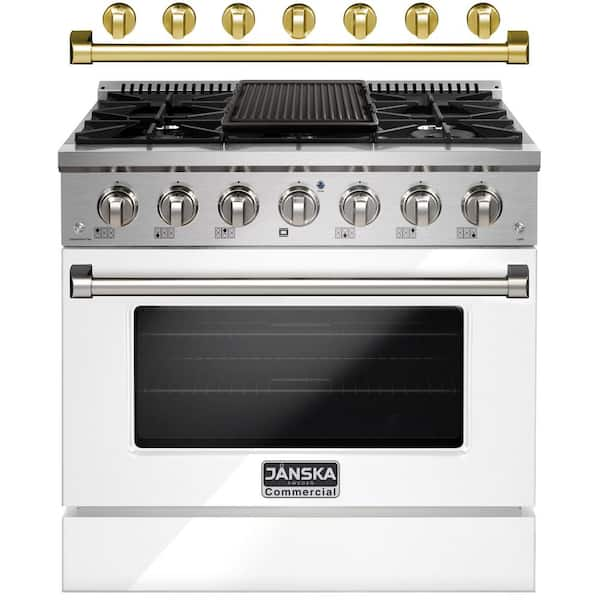This image features a sleek, modern stove and oven combination, predominantly in stainless steel. The large picture showcases a Janska Commercial brand appliance, with the brand name "JANSKA" displayed in gray, all-capital letters against a black rectangular background, and "COMMERCIAL" in black letters against a gray background located on a small rectangle beneath the oven window. The oven door stands out with a slightly lighter shade of silver compared to the stovetop. A prominent silver handle runs across the top of the oven door, just below seven burner control knobs situated on the front face.

The stovetop is clearly a gas burner model, with four burners and a central skillet area, all housed in a sleek black surface. Above the stove, there's an unattached gold-colored bar, possibly mounted on the wall, which features additional gas burners. This bar appears to be illustrating an available customization option with gold colored burner knobs and accents, offering a visual contrast to the silver knobs and handle seen on the primary appliance. The overall look of the stove is shiny and new, reflecting its contemporary and sophisticated design.